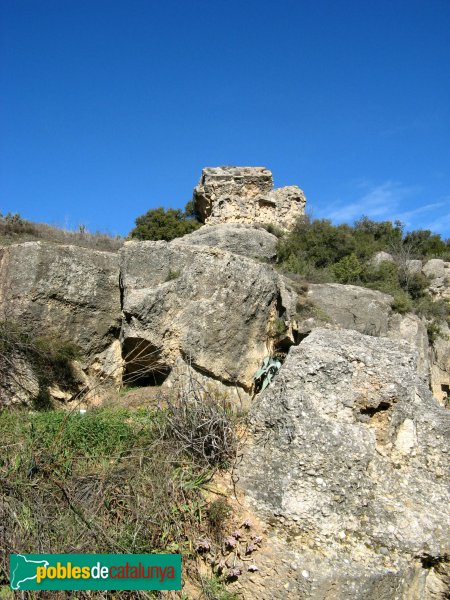The photograph captures a rugged hillside dotted with large rocks ascending a gentle slope. Prominently featured in the lower right corner of the foreground is the closest large rock, surrounded by patches of short grass interspersed with brown weeds and a bush. Directly above, the hillside becomes steeper with more large rocks, including a standout formation that appears as though it might be crowned by a flat-topped stone structure. To the left and right of this central rock cluster, scraggly bushes and additional rocks pepper the landscape. The top third of the image is dominated by a brilliant blue sky.

In the bottom left-hand corner of the photograph, there is a green rectangular label reading "Pobles de Catalunya" with "Pobles" in yellow, "de" in white, and "Catalunya" in red. A white outline of a map accompanies the text.